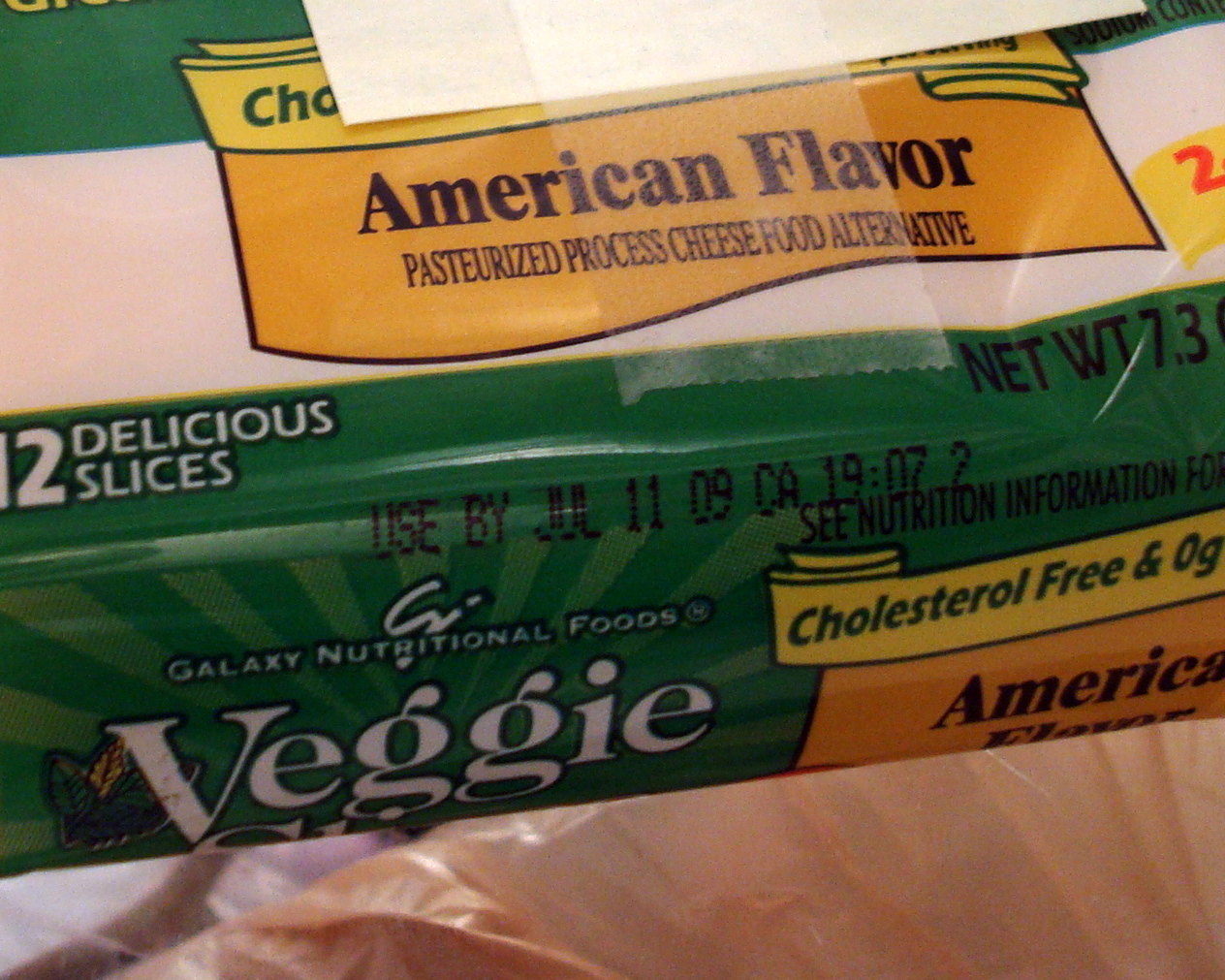This image depicts the packaging of an American-flavored pasteurized processed cheese food alternative. The package is predominantly green, accented with yellow highlights designed to emphasize the American flavor. The product is branded as "Veggie Slices" and is manufactured by Galaxy Nutrition Foods. Notably, the packaging specifies a use-by date of July 11, 2009. The image prominently features two mouth-watering slices of the cheese food alternative, suggesting its appeal and usage.